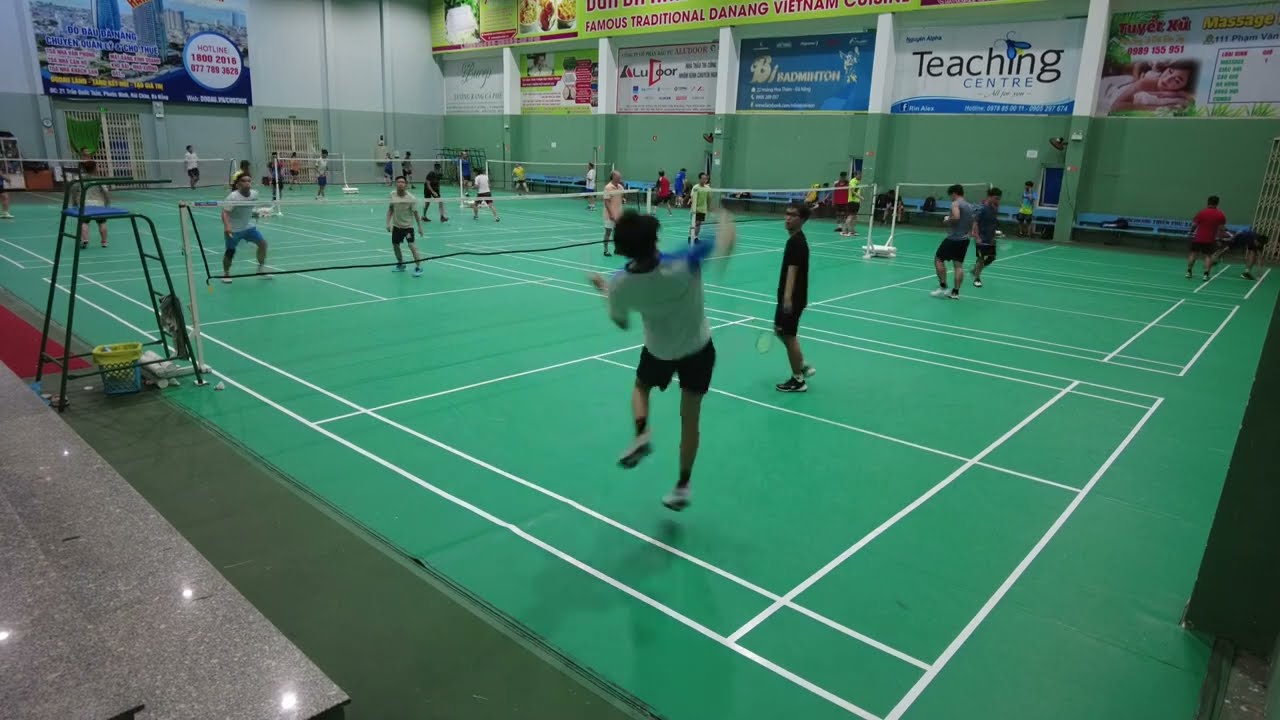In the image, a bustling indoor facility with pale green courts lined in white hosts numerous players engaged in lively badminton matches. A central player is captured mid-hit, while around 20 others, dressed in a variety of colors such as white, black, salmon, red, and gray, are scattered across six distinct courts, each sectioned off with low-hanging nets resembling volleyball nets. To the left of the image, an umpire’s chair stands on one of the courts, overseeing the dynamic scene. The background wall, part of what appears to be a multi-purpose room, features tall pillars adorned with colorful advertisement banners in blues, reds, whites, greens, and yellows. These advertisements include messages for a teaching center, massage services, and a partially visible banner mentioning "famous traditional" cuisine, hinting at an international setting. The entire setting is vibrant and bustling, capturing a recreational atmosphere filled with enthusiastic badminton players.